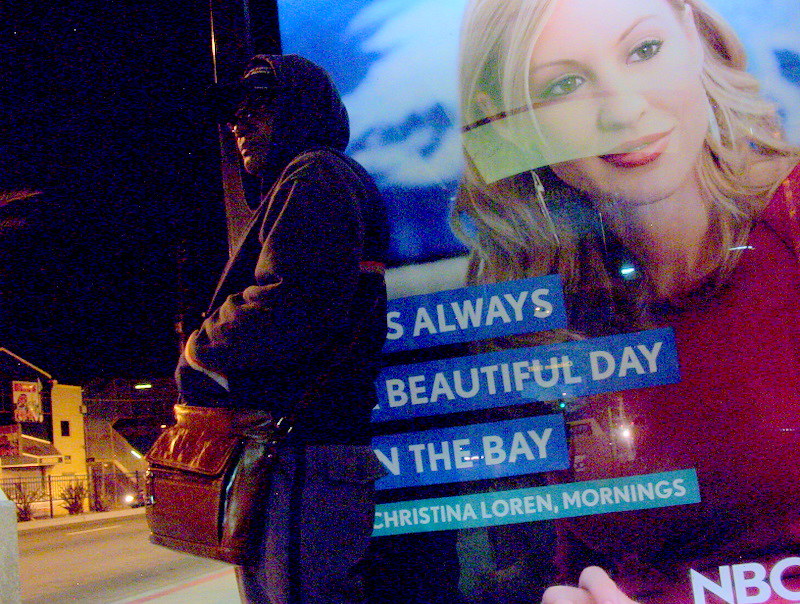The photo, taken at night, features a man standing left of center on what appears to be a street or near a bus stop. He is dressed in dark, potentially American Postal Service attire that includes a hooded sweatshirt folded over a baseball cap and dark pants with a stripe. He carries a brown, briefcase-sized shoulder bag across his front and wears sunglasses. The man is leaning against a large advertisement for an NBC newscast, prominently displaying a blonde woman in a red top against a blue background. The text on the ad reads, "Always a beautiful day in the Bay. Christina Lauren Mornings," with an NBC logo in the bottom right corner. The image also shows buildings and a completely black sky in the background, with some reflection present on the surface of the advertisement.